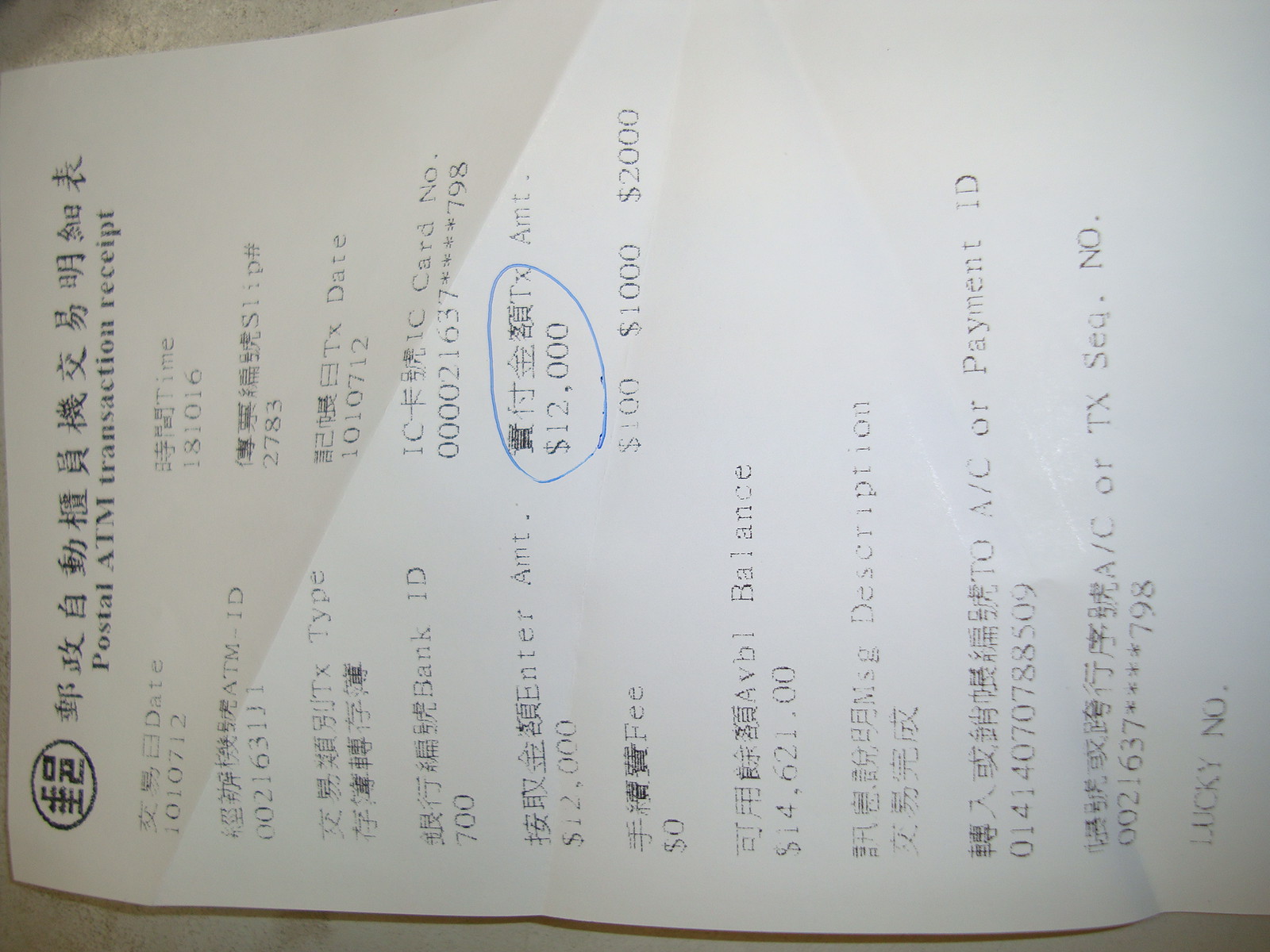The indoor color photograph depicts a printed receipt on white paper with black text, lying sideways on what appears to be a marble counter. The image is turned 90 degrees to the left, requiring viewers to tilt their heads for proper reading. The receipt features a combination of Asian characters and English text. At the top, it states "Postal ATM Transaction Receipt." The date of the transaction is January 7th, 2012 (noted as 10-10-7-12), and the time is recorded as 18:10:16. The central part of the receipt prominently displays an amount of $12,000, although it is not clear whether this amount was withdrawn or deposited. Below this amount, it lists additional denominations of $100, $1,000, and $2,000. The available balance in the account is shown as $14,621. No transaction fee is mentioned, and towards the bottom, there are details including a payment ID and a note indicating “lucky number.” The receipt is clearly legible and well-lit, yet it is still difficult to determine the exact nature of the transaction.